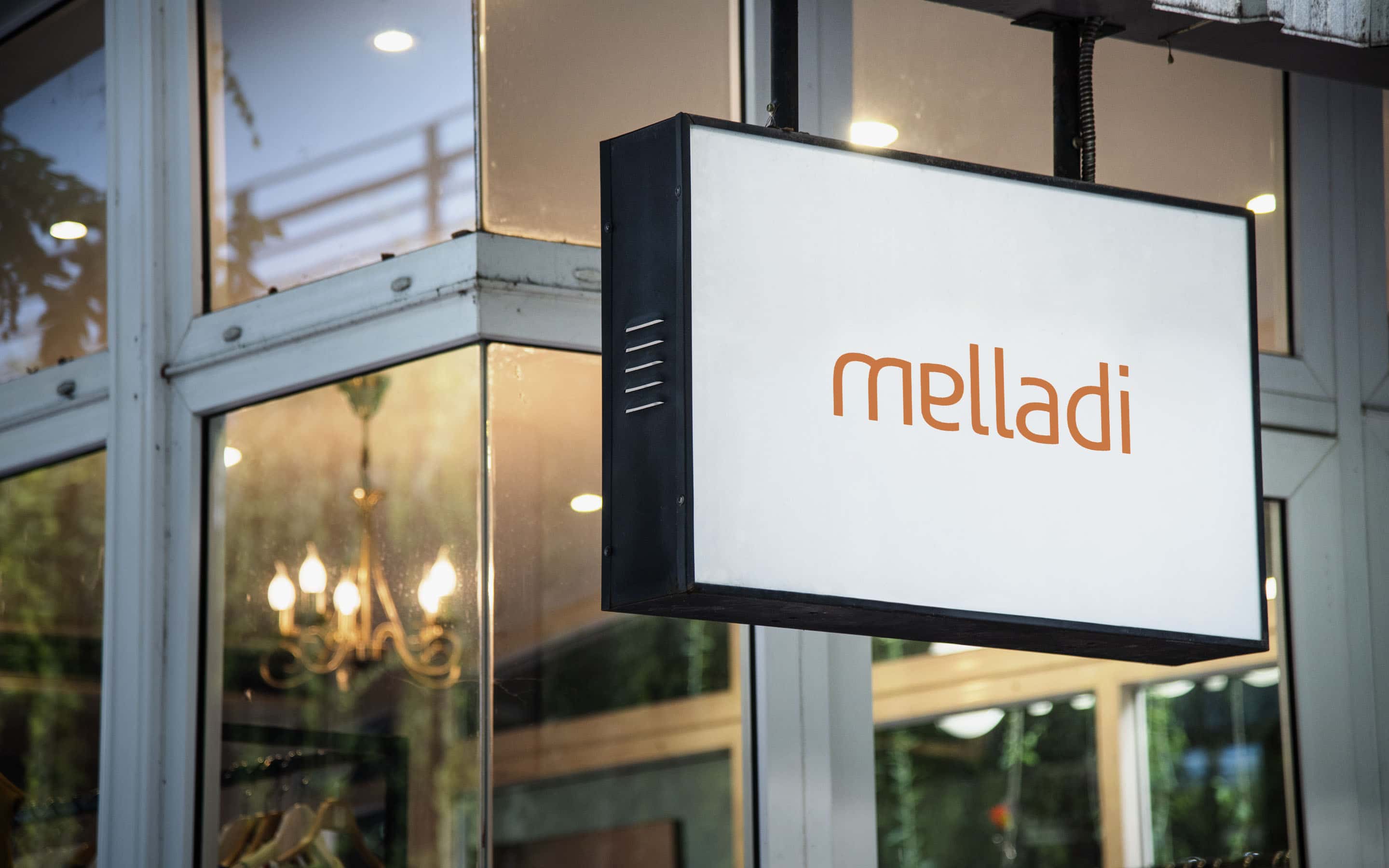The photo was taken outdoors, looking into a corner of a building with large, prominent windows framed in a light gray or off-white color, possibly indicating a business in a city. Suspended from the ceiling above one of the windows is a thick, black-framed sign with a white surface. The sign displays the word "Maladi" or "Miladi" in a unique, modern orange font. The edges of the building's structure feature a sturdy metal frame. Through the windows, a gold-colored chandelier with lit bulbs is visible, casting a light yellow glow on the interior. Additional spotlights add to the illumination, suggesting it might be either day or night. The interior walls appear to be a soft blue, and there's a coat rack with some empty hangers in one of the bottom windows. Some greenery can be seen reflecting from across the street, adding to the urban ambiance of the scene.